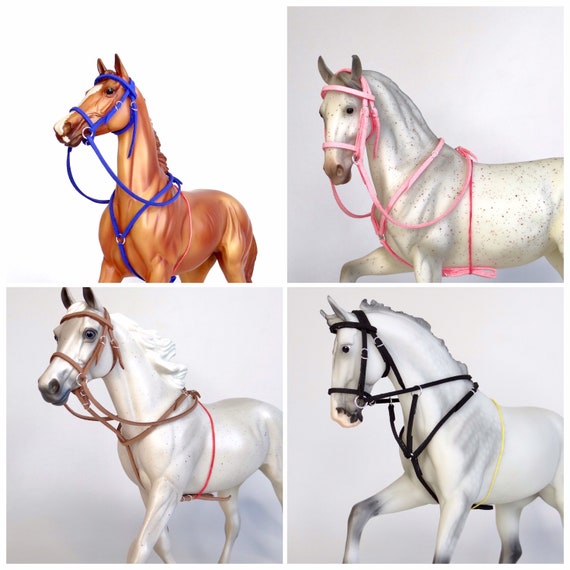The image is a collage composed of four zoomed-in photos of toy horses, each occupying one quadrant in a grid style. The top left quadrant features a brown horse with a defined musculature, adorned with a blue bridle that wraps around its mouth, face, neck, and chest. This horse's head is in profile, facing left. The top right quadrant presents a white horse with brown flecks and a light brown muzzle, wearing a pink bridle and lifting its right front foot slightly. In the bottom left quadrant, another white horse is depicted with flowing white hair, striding to the left with its left front leg extended. It wears a brown bridle. Lastly, the bottom right quadrant shows a white horse with gray shadings on its coat and legs, wearing a black bridle and also raising its right front foot. Each horse is depicted from the body upward, including the neck, head, and part of the legs, with the bottom portions of the legs cut off.